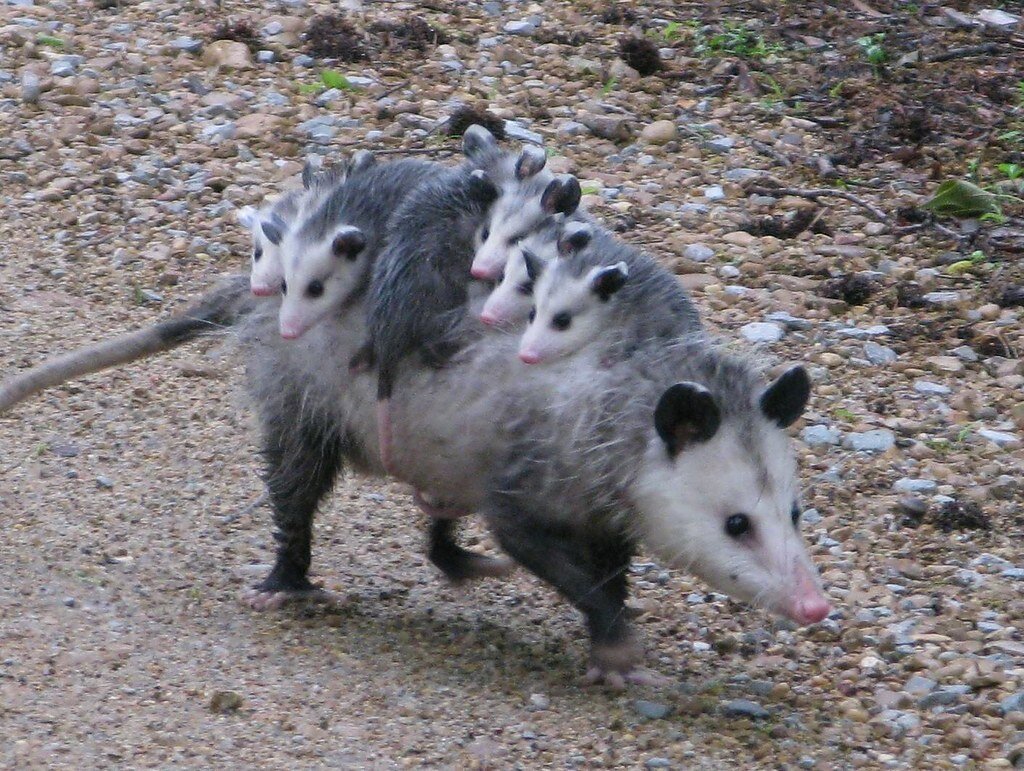In this detailed wildlife photograph, a large possum with a pink nose, dark black ears, and eyes, stands out with its white face and white-gray fur as it traverses a gravel road covered in varying sizes of pebbles. In the foreground, the small, light-colored pebbles gradually shift to larger, darker ones, creating a textured backdrop. Riding on the possum's back are six baby possums exhibiting similar features: white faces, pink noses, and black eyes. The first three babies near the neck face outward to the left, while another, positioned in the middle, faces the opposite direction with only its gray body and a pink tail visible. The remaining two babies align with the first group, also facing left. The adult possum, with its slender pink nose and white belly, is walking towards the right side of the image, showing distinct black legs and gray neck fur beneath its hairy, somewhat spiky-textured body, creating a rich contrast against the gravel road.